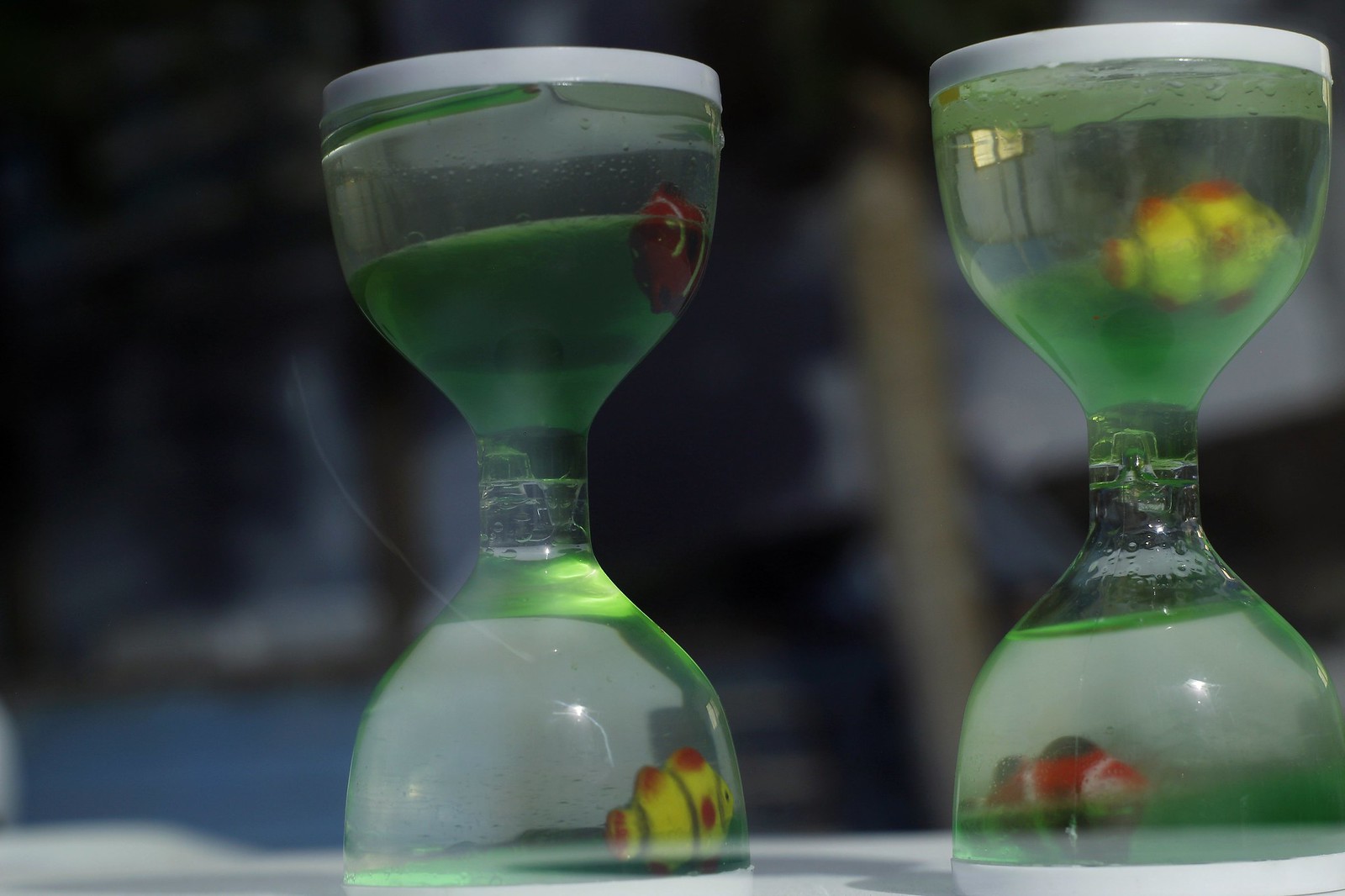This close-up color photograph in landscape orientation features two hourglass-shaped containers, likely made of plastic, designed to resemble wine glasses fused together. Each container is filled with liquid, exhibiting a greenish-white tint particularly noticeable at the top and bottom sections. The containers are sealed with white caps at both ends. Inside each compartment of the hourglasses, there are small fish that could be real or fake. On the bottom left of the first hourglass, a fish is yellow with orange fins, black stripes, and a small red stripe on the side. The top left fish is red with white stripes and black blotches. On the bottom right, a fish sports red with white stripes and black spots on its fins, while the top right fish is yellow with orange around its fins and black stripes. The clear glass of the hourglasses creates a bubbly effect where they join. All this is set against a blurred background featuring indistinct shelves and a collage of colors including black, blue, tan, and white, enhancing the focus on the unique hourglass containers and their occupants.